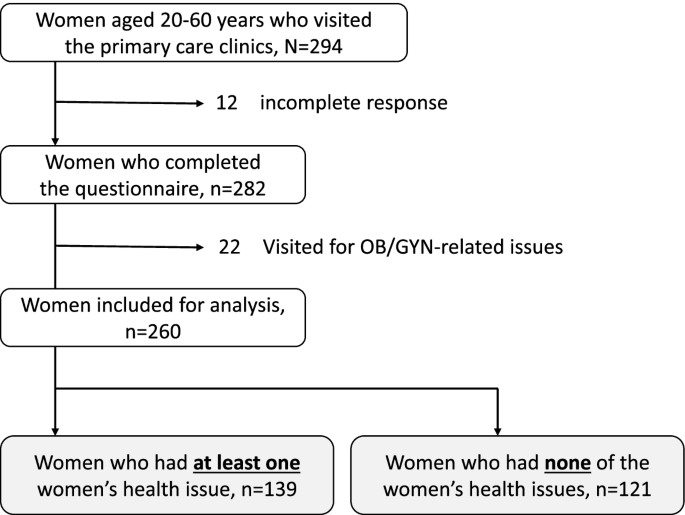This diagram illustrates the analysis of women aged 20-60 years who visited primary care clinics. Starting with an initial group of 294 women, the flowchart details their progression through the study. Initially, 12 women were excluded due to incomplete responses, leaving 282 who completed the questionnaire. Subsequently, 22 women who visited for OB-GYN-related issues were also excluded, resulting in a final sample of 260 women for analysis. This final group is then divided into two subgroups: 139 women who had at least one women's health issue and 121 women who had none of these issues. The diagram utilizes arrows and square boxes, with the final two subgroups highlighted in a gray background to distinguish them from the rest.